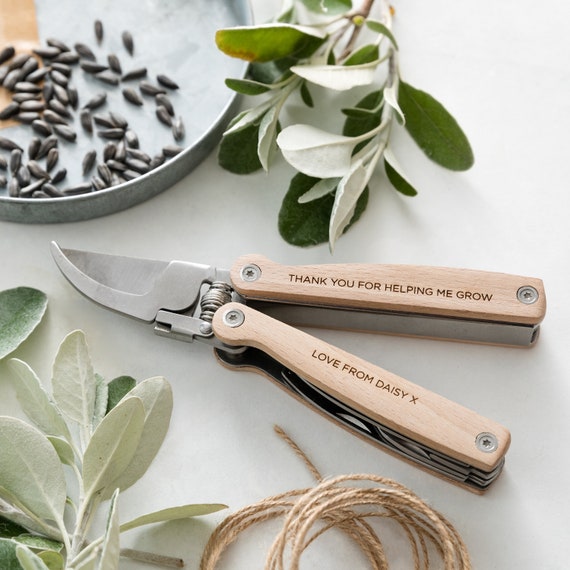The image features a white, well-lit surface with a collection of gardening items artfully arranged. At the center, there's a high-quality multi-tool with wooden handles, which also serves as pruning shears or clippers. The tool is etched with the message, "Thank you for helping me grow. Love from Daisy X." Surrounding the clippers are various gardening elements: to the upper left sits a small metal tray filled with black seeds; to the right, there are green and white leaves attached to thin stems. Just below the shears is a spindle of brown twine, which could be used for tying the plants or simply as decoration. Additional leaves can be seen at the bottom left corner. The entire scene casts soft shadows, adding depth to the simple yet elegant arrangement.